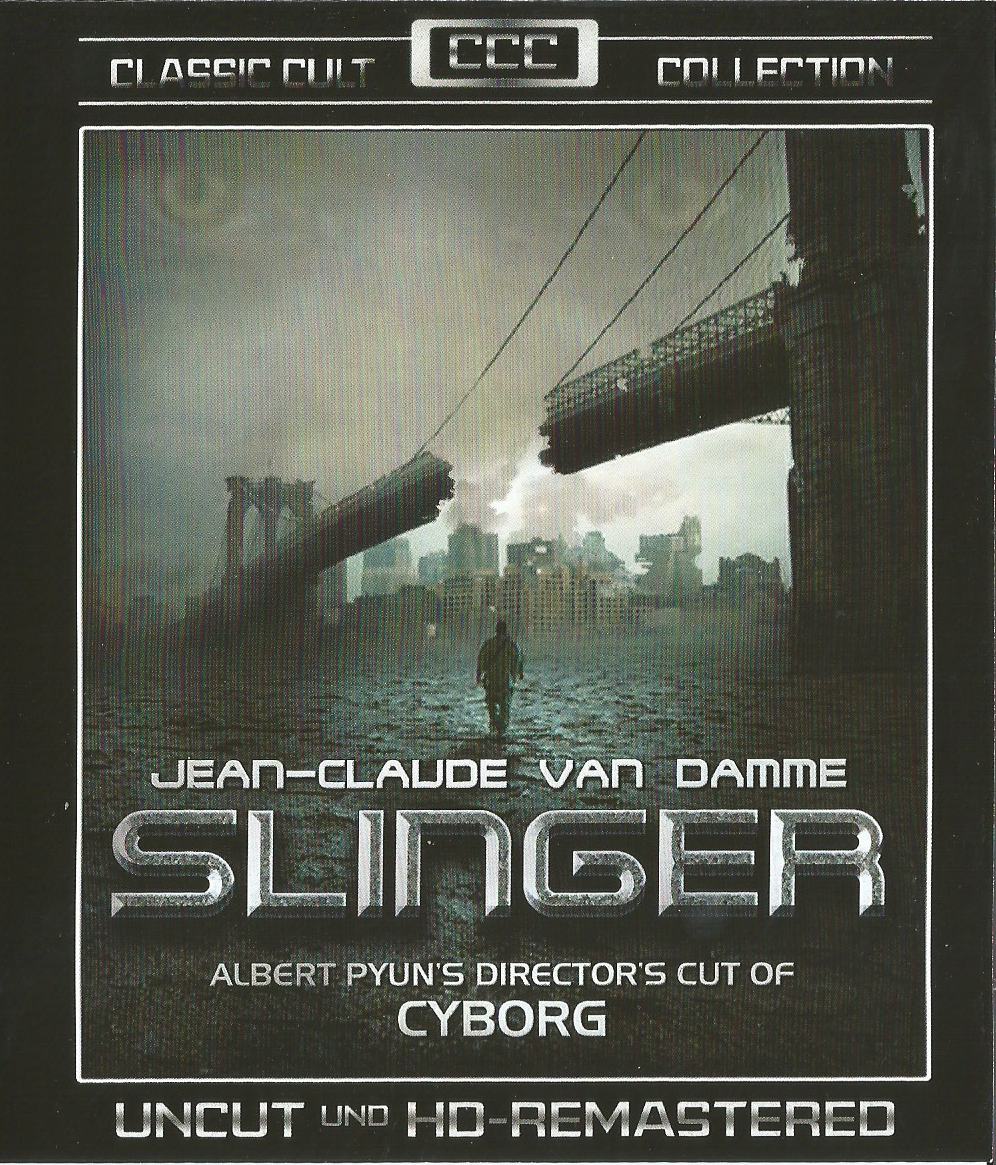The image, in portrait view, appears to be a movie poster or the cover for physical media. The top portion of the poster features a black background with silvery white letters that read "Classic Cult Collection" flanking the "CCC" logo. Dominating the center of the poster is a striking visual of a man, identified as Jean-Claude Van Damme, walking on water beneath a large suspension bridge. The bridge, which looks similar to the Brooklyn Bridge, has a significant section missing. In the background, a possibly Manhattan cityscape rises ominously with hues of blacks, dark blues, and whites, enhancing the dystopian atmosphere. Above the cityscape, the sky is subtly filled with the ghostly image of giant eyes, giving the impression of an unseen watcher overseeing the scene. Towards the bottom of the image, bold white text states, "Jean-Claude Van Damme, Slinger, Albert Pyun's Director's Cut of Cyborg," followed by "Uncut and HD Remastered." This meticulously detailed poster invokes a sense of mystery and intrigue, characteristic of classic cult films.